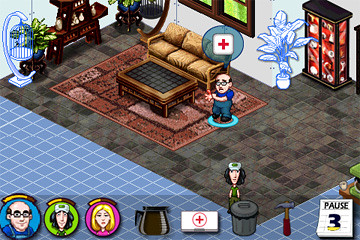In this pixelated scene from a retro-style video game, the square image depicts the interior of a living room with distinct design elements. The bottom portion features a floor covered in small light and dark gray tiles, arranged in a neat grid pattern. Adjacent to this, there is a large red patterned rug that acts as a cozy accent piece. Placed on the rug is a brown couch and a matching brown coffee table with a sleek black top.

The floor surrounding the rug is covered in blue and gray tiles with white mortar, creating a visual boundary between the two different flooring types. In the center of the living room stands an avatar: a balding man wearing horn-rimmed glasses, a white shirt, and blue pants. Hovering above his head is a blue speech bubble containing a white box emblazoned with a red cross, suggesting some sort of medical information or alert.

In the lower portion of the image, additional avatars can be seen, adding to the dynamic and interactive atmosphere of the game scene.